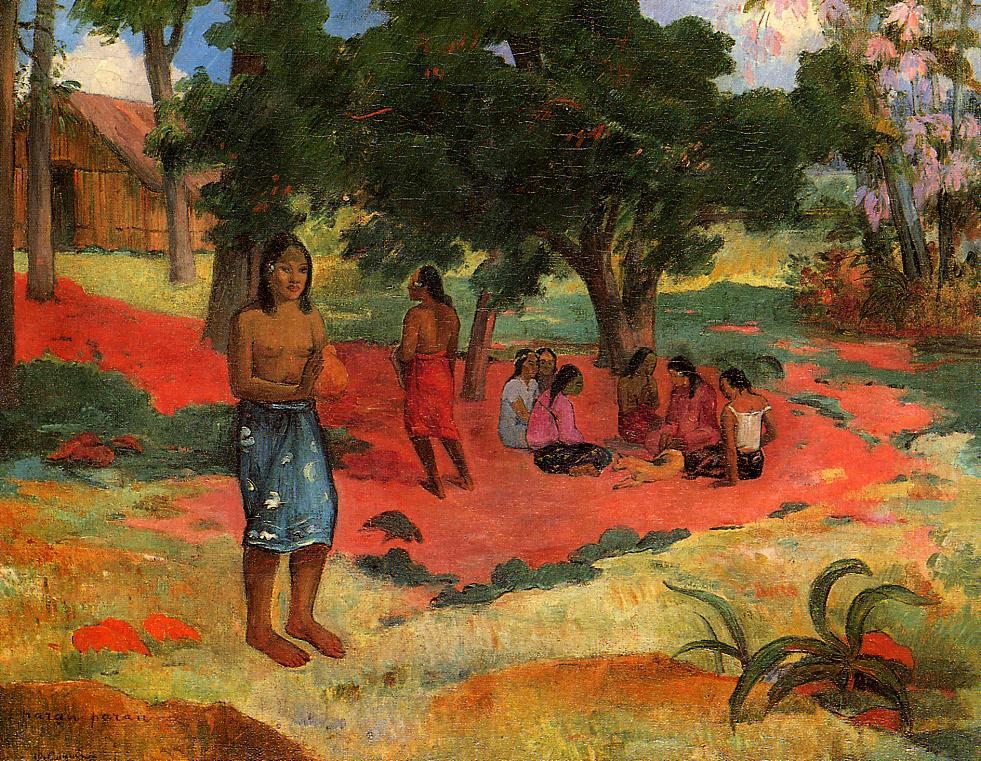This painting, attributed to Paul Gauguin, captures a vibrant daytime scene featuring Indigenous individuals in a natural setting. Dominating the foreground is a topless, brown-skinned woman with black hair adorned by a white flower behind her right ear. She stands gracefully, holding a clay object in her hands, and wears a blue skirt with a white pattern, her feet planted firmly on the green grass. Behind her, slightly to the left, stands another woman with her back turned, draped in a red wrap around her lower legs, contrasted against the reddish soil beneath her feet.

At the heart of the scene, a circle of Indigenous women, some topless and others fully clothed, sit on the red-tinted ground beneath the shade of several trees, accompanied by a brown dog with a distinctive black spot. These trees are shorter and have wide, white-topped canopies. Flanking the central group are two distinct types of trees; on the far left, trees stand tall near a hut with wood or reed siding and a slanted grass roof, almost hidden amongst the foliage. On the far right, trees with purple and pink-tinged branches reach upward.

The painting employs striking contrasts of green grass in the sun and darker green in the shade, with rich, warm tones of the ground adding depth. Despite the faded artist’s name on the bottom left, the signature style of Gauguin imbues the scene with a sense of serene, yet dynamic, everyday life in an Indigenous island community.